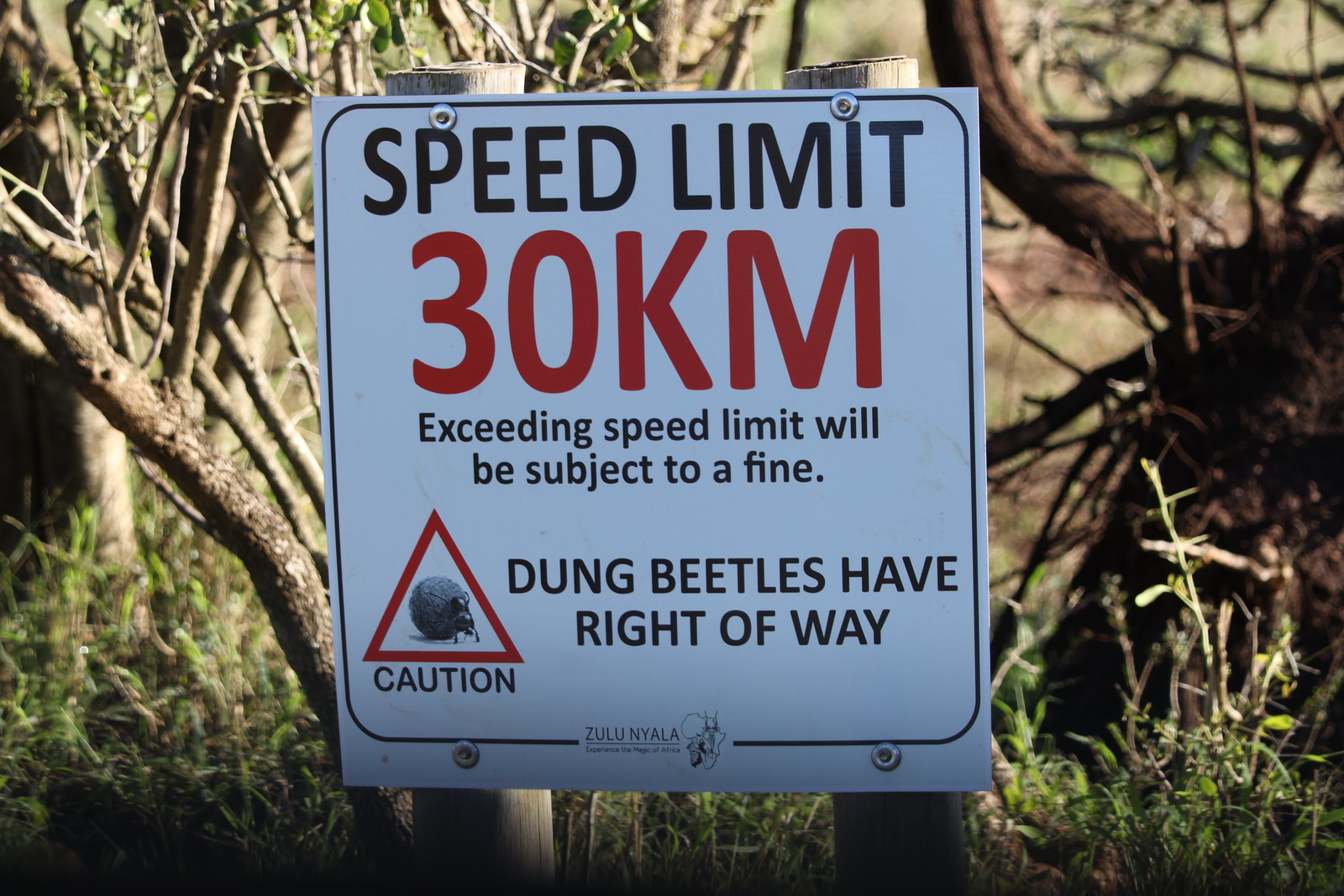This landscape photograph, captured in a forested area with trees, branches, and leaves forming the background, features a distinct sign held up by two wooden poles. The white sign, secured with bolts, displays a clear warning and message. At the top, the words "SPEED LIMIT" are written in bold black letters, followed by the prominent red text "30 kilometers" — the largest text on the sign. Below, in black, it states, "Exceeding speed limit will be subject to a fine." To the left, within a red triangle, is the image of a dung beetle pushing a ball of dung, accompanied by the word "CAUTION" in black underneath. Adjacent to this, it reads, "Dung beetles have right of way" in black letters. At the very bottom, the text "Zulu Nyala" is displayed next to a logo featuring the outline of Africa with some imagery on it. The sign serves both as a speed warning and as a reminder to respect the local dung beetles vital to the ecosystem in this wilderness setting.